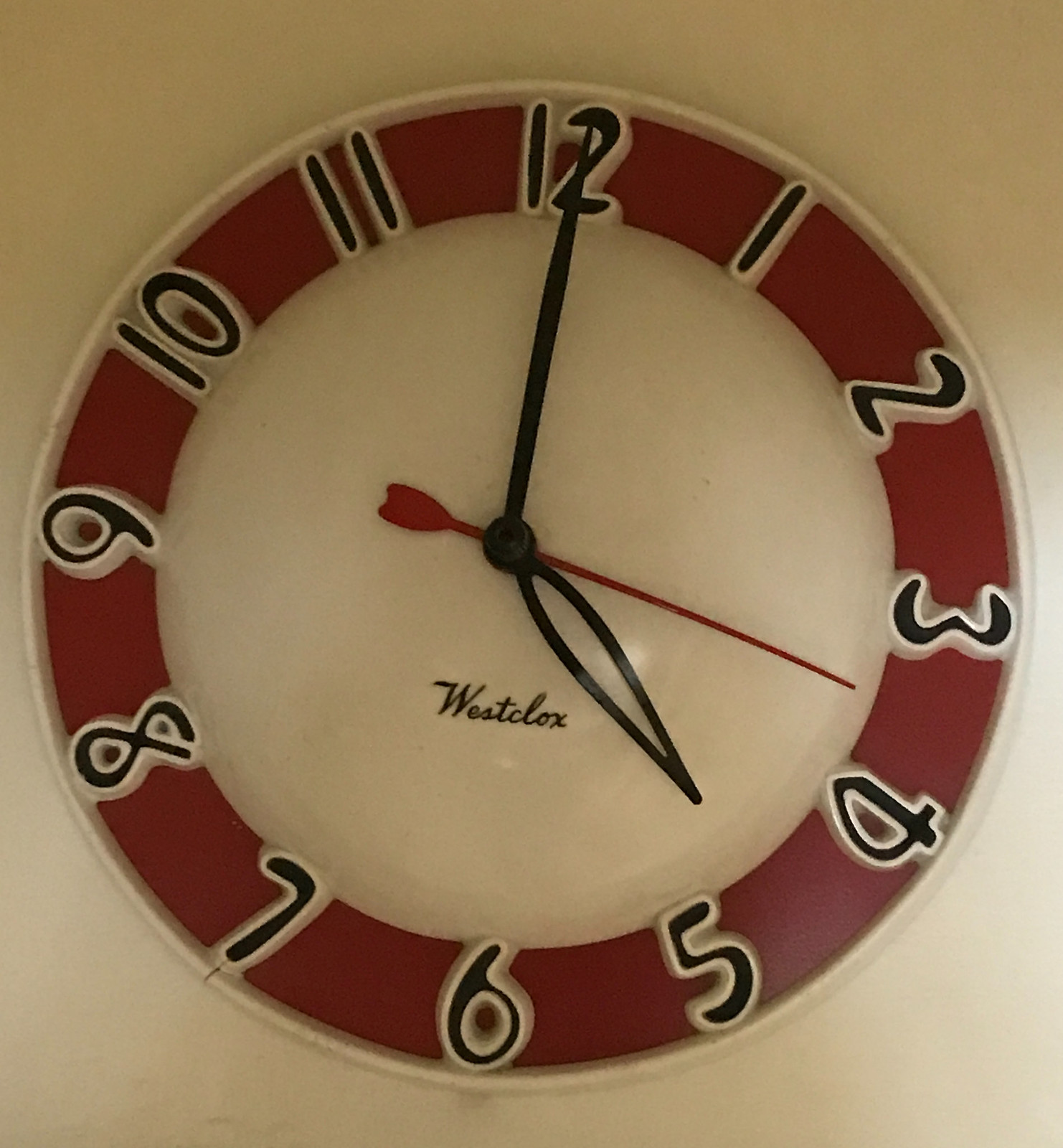A vintage-style clock is prominently featured against a smooth white wall. The clock’s design boasts a perfectly round shape with a distinctively minimalist central white circle. From the middle of this circle, three clock hands extend outward: a slender red second hand, a longer and thicker black minute hand, and a shorter, wider black hour hand. Directly beneath the intersection of these hands, "West Clocks" is elegantly scripted in black cursive text. Encircling the plain white center is a vivid red border, also circular, that houses bold black numbers indicating the hours. Each number is characterized by a playful, cartoonish font, further emphasized by a contrasting white outline that enhances readability and adds to the clock’s whimsical aesthetic.